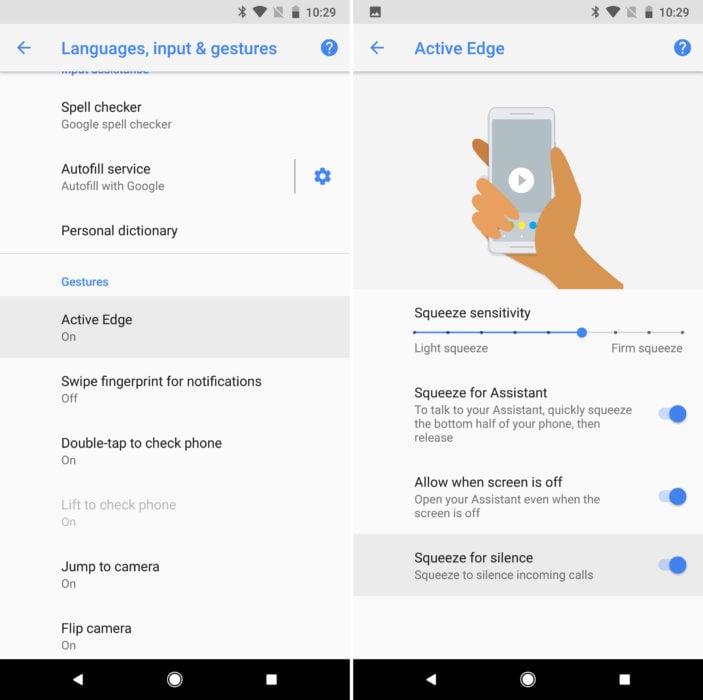**Image Description:**

The image features side-by-side screenshots from a mobile device, each showing different settings and options.

**Left Screenshot:**

- **Status Bar:** The top bar is light gray, displaying icons from left to right: Bluetooth, Wi-Fi, an unknown gray icon with a diagonal line, battery (approximately 50%), and the time (10:29).
- **Main Interface:**
  - A blue left-pointing arrow and the text "Languages, Input, and Gestures" in blue.
  - A blue circle with a white question mark next to it.
  - Below, a list of options with black text:
    - **Spell Checker:** Black text with "Google Spell Checker" in gray.
    - **Autofill Service:** Black text with "Autofill with Google" in gray.
    - **Personal Dictionary:** Black text with a blue gear icon to its right.
  - A gray line separates the sections.
  - **Gestures Section:** In blue text.
    - **Active Edge:** Marked as "On."
    - **Swipe Fingerprint for Notifications:** Marked as "Off."
    - **Double Tap to Check Phone:** Marked as "On."
    - **Lift to Check Phone:** Faintly marked as "On."
    - **Jump to Camera:** Marked as "On."
    - **Flip Camera:** Marked as "On."
- **Bottom Bar:** Black with three icons: a white play triangle pointing left, a white circle in the middle, and a white square on the right.

**Right Screenshot:**

- **Status Bar:** Identical to the left screenshot with top bar light gray, same icons (Bluetooth, Wi-Fi, unknown gray icon with a diagonal line, battery at 50%, and time at 10:29).
- **Main Interface:**
  - **Section Title:** "Active Edge," capitalized and in blue, with a left-pointing arrow and a blue circle with a white question mark.
  - **Image:** A hand holding what appears to be an iPhone with a play symbol below it.
  - **Squeeze Sensitivity Section:**
    - Labeled with a horizontal point graph marked "Light Squeeze" on the left and "Firm Squeeze" on the right.
    - The slider is positioned at the sixth position from the left towards the "Firm Squeeze" end.
  - **Squeeze for Assistant:**
    - Instruction to "talk to your assistant quickly, squeeze the bottom half of your phone, then release." This option is activated and blue.
  - **Allow When Screen is Off:**
    - Option to "open your assistant even when the screen is off," activated and blue.
  - **Squeeze for Silence:**
    - Option to "silence incoming calls" by squeezing, activated and blue.
- **Bottom Bar:** Black with three icons identical to the left screenshot: a white play triangle pointing left, a white circle in the middle, and a white square on the right.

This detailed description thoroughly captures the various elements and settings displayed in the two screenshots.